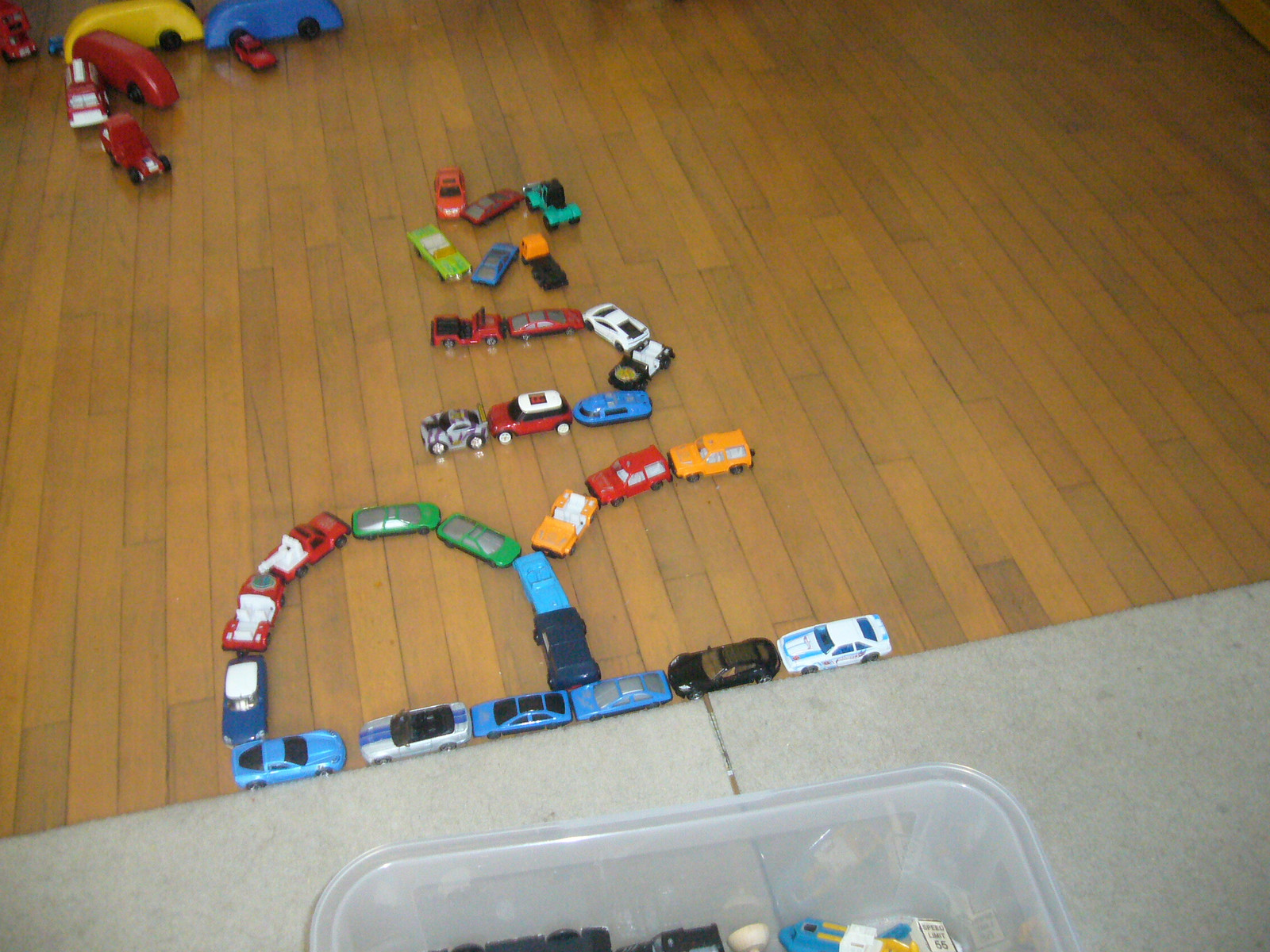This vibrant image captures a playful scene on a light brown wooden floor with small floorboards, accented by partially visible gray carpet pieces. At the heart of the scene are an array of colorful toy cars, predominantly Hot Wheels, which have been meticulously arranged in a whimsical formation spelling out "RUSS." These cars showcase a vivid color palette including shades of orange, red, yellow, green, blue, white, navy, brown, and silver, and include various models such as sports cars, hot rods, police cars, trucks, and semi-trucks.

In the upper left corner, there's an opaque plastic tub overflowing with more toys, hinting at the promise of extended playtime. Notably, there are also larger toy vehicles, including die-cast and wooden cars, showing broader black wheels and curved, windowless designs in primary colors like red, yellow, and blue. Alongside these, there are red die-cast firetrucks and trucks, adding to the vibrant assortment.

This beautifully organized chaos on the floor clearly captures the aftermath of a child's imaginative playtime, with some cars forming a complete half-moon shape, while others remain scattered or partially arranged. The presence of a white folding table at the bottom of the image and a light gray couch slightly out of frame offers a comforting backdrop to this colorful tableau.